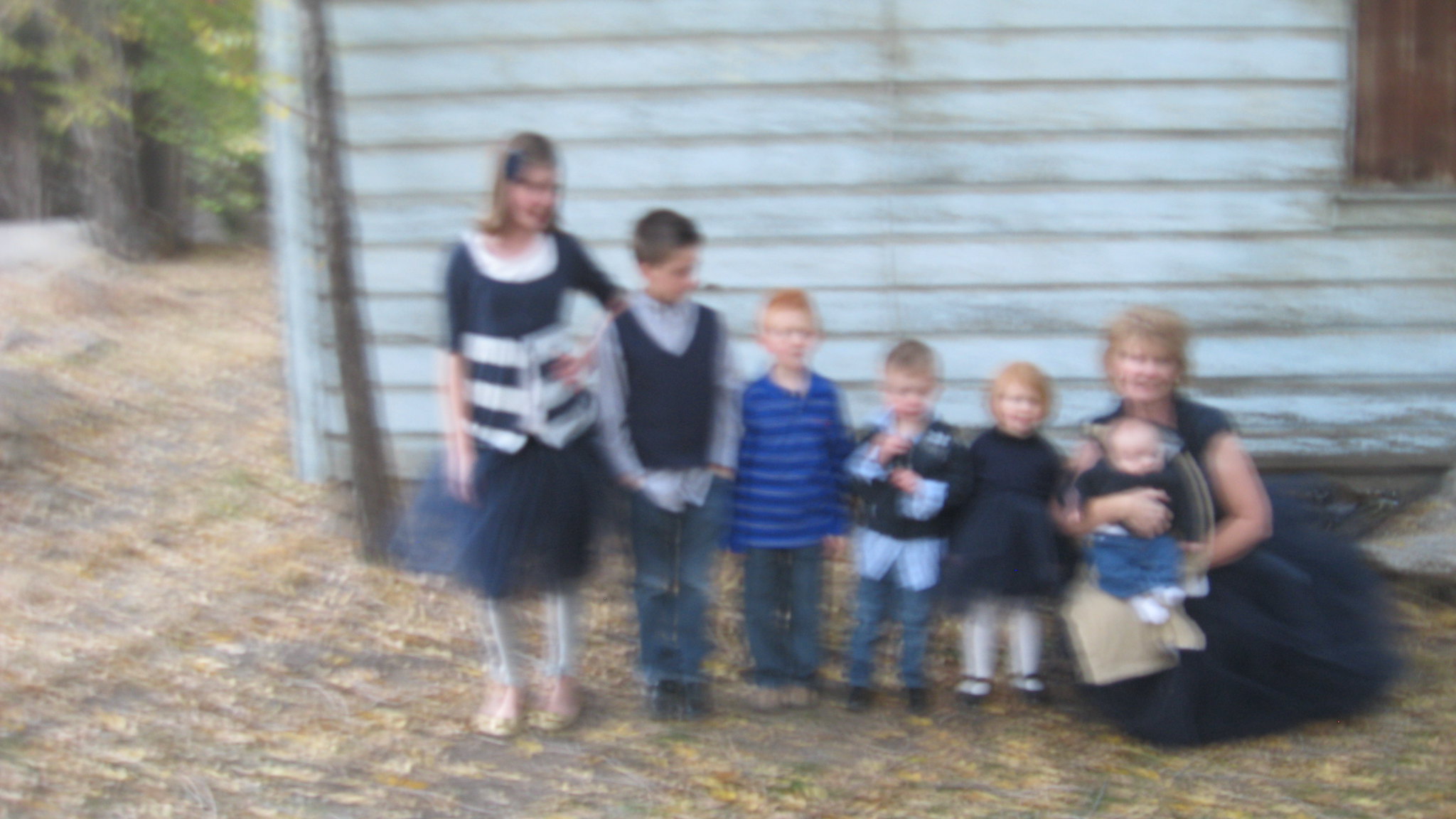In this autumnal scene, an elderly woman sits serenely on the right, attired in a blue dress and cradling a baby in her arms. The ground beneath them is carpeted with brown earth and an array of scattered, colorful leaves, suggesting a fall setting. To the left of the woman, a line of children stretches out, each progressively taller than the one before. 

First in line, standing closest to the woman, is a young redheaded child dressed in a dark blue blouse. Next is a slightly older child, donning a black and light blue striped shirt paired with jeans. Following this child, another redhead is seen wearing a blue shirt and orange jeans. Continuing the height progression, a taller youth appears in a gray and black shirt. At the far left end of the group, a young girl in a black dress stands poised. The entire group is positioned in front of a white wooden house, adding a rustic, homely backdrop to this charming portrait.